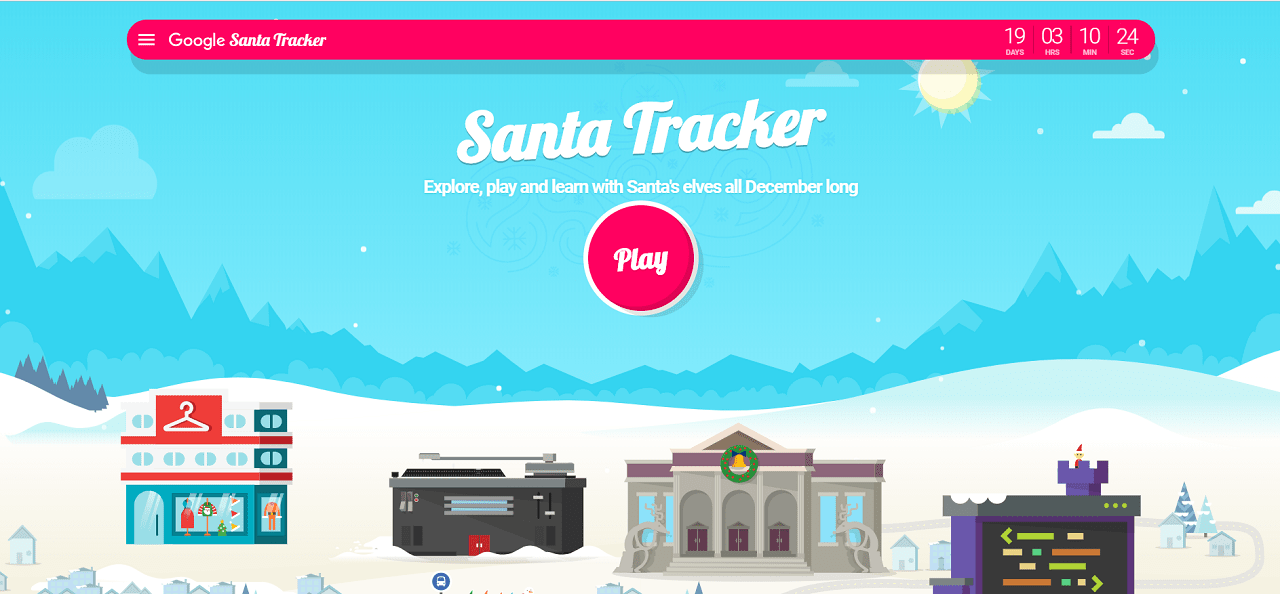This screenshot displays the interface of a Google Santa Tracker, designed to follow Santa Claus's journey. The scene is set in a picturesque, snowy mountainous area. Dominating the top center of the screenshot is a long, oval-shaped bar with a red background. In white font, it prominently reads "Google Santa Tracker." The tracker indicates that there are "19 days, 03 hours, 10 minutes, and 24 seconds" remaining until Santa's arrival. Diagonally printed at the top center of the screen, the phrase "Santa Tracker" ascends towards the right, followed by a tagline that reads, "Explore, Play, and Learn with Santa's Elves all December long." Positioned below this tagline is a red circle outlined in white, with the word "Play" written in white at its center, inviting users to engage with the tracker’s interactive features.